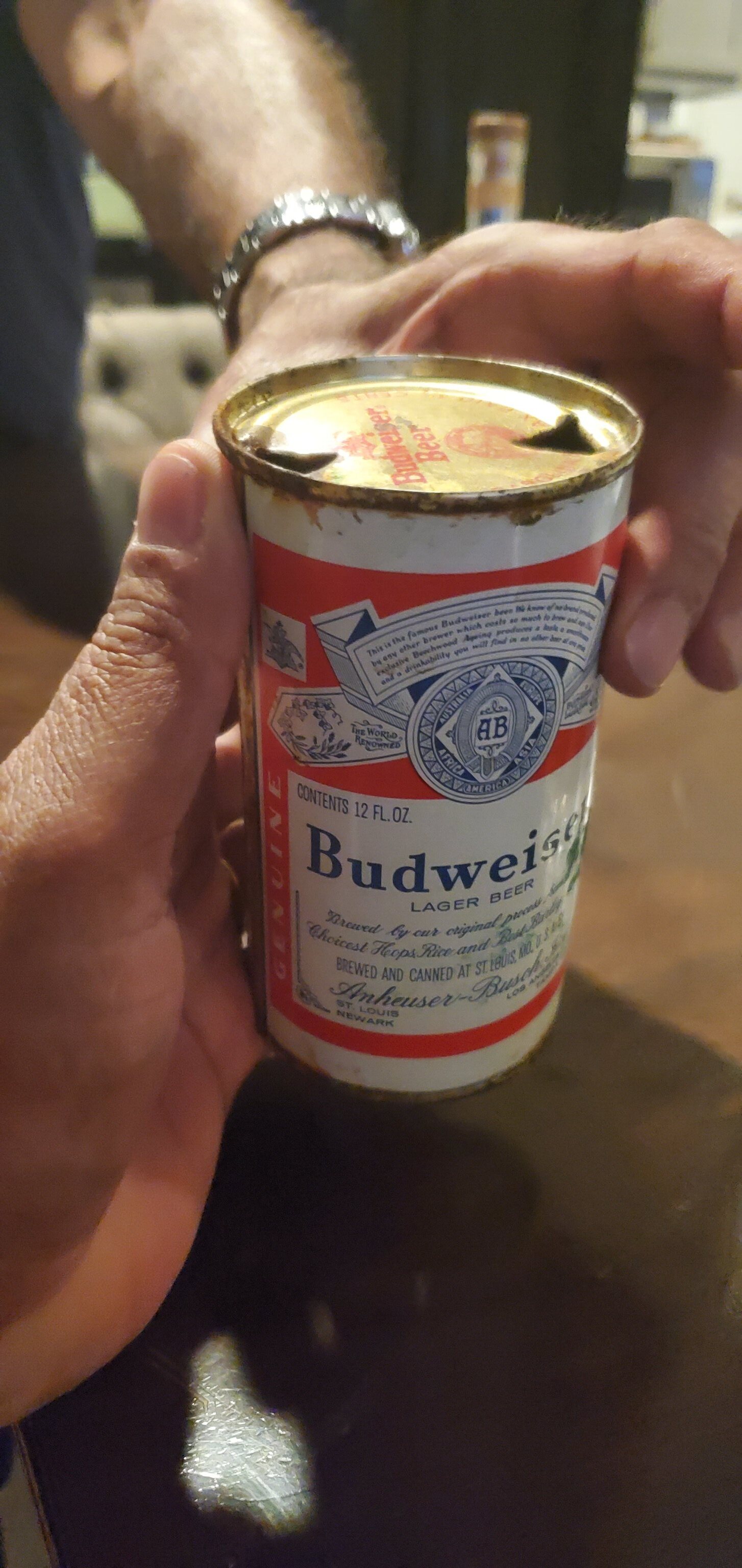A close-up, vertical photograph captures a moment frozen in time where one hand extends an old Budweiser can to another. The can itself is a vintage artifact, showcasing a white background with an orange banner wrapping around it, adorned with the iconic blue Budweiser text and logo. Unlike the modern snap-top cans, this one features two triangular holes at the top, indicating that it was opened with a can opener, a relic from a bygone era. The can fits snugly in the hand, suggesting it's slightly larger than a grown man's palm. Time has etched its mark, as evident from the rust encircling the top and bottom of the can, adding a layer of historic charm to the scene.